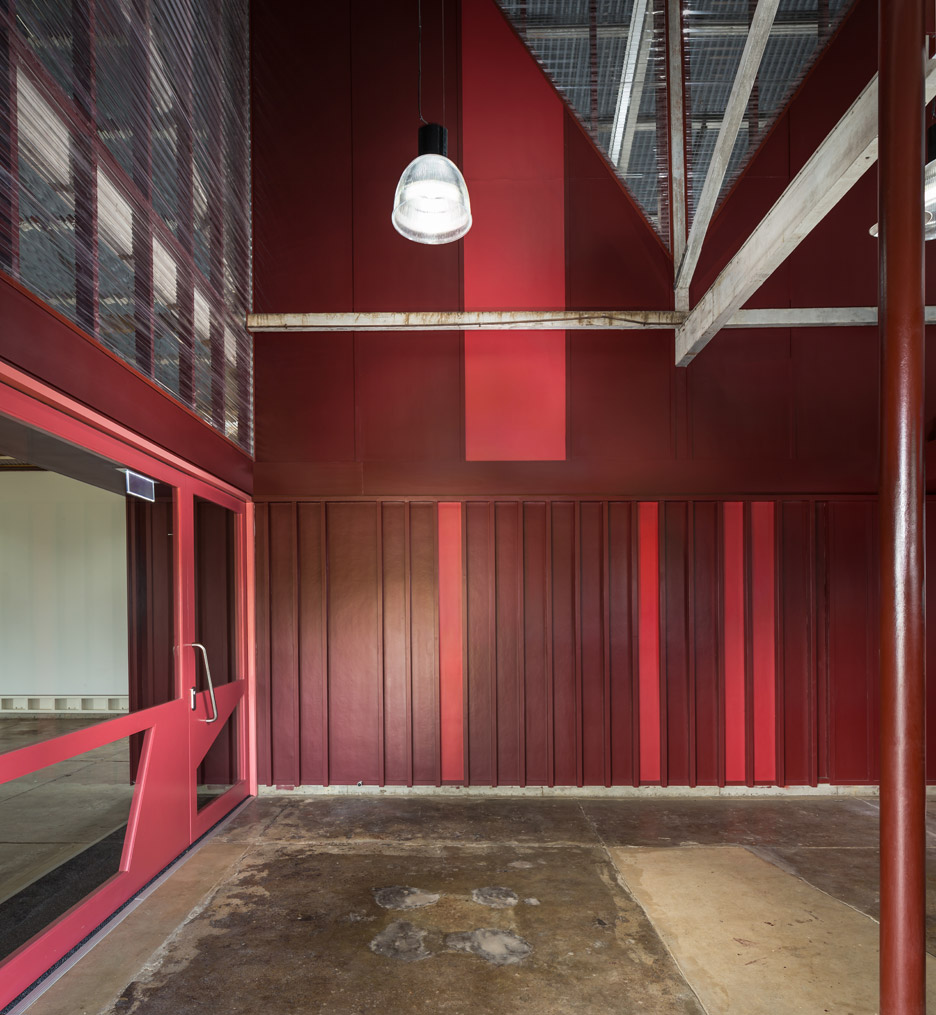The photograph depicts the interior of a contemporary garage-like space. The flooring is concrete, stained in places to produce a dark brown appearance on the otherwise tan surface. The walls are paneled with vertical siding in shades of burgundy and red, featuring occasional red stripes, creating a striking visual effect. The structure of the building includes scaffolding made from either aluminum or steel overhead. 

A prominent maroon-painted pillar divides the space, and a large white light with a black base hangs from the ceiling above the left bay. Adjacent to this area, the left wall features a significant amount of glass, framed by painted red metal, leading to a room that could be an office or another part of the building. The glass door on this wall has a modern silver-tone handle and opens into an area with another concrete floor and white walls.

Above this glass-enclosed section, the second floor is visible, along with ceiling lighting through the overhead beams. The ceiling features mesh metal that might cover attic space or vents, adding to the modern industrial aesthetic of the space. 

Overall, the detailed combination of stained concrete, colorful paneling, and mixed-use of modern materials creates a dynamic and contemporary environment, rich in visual interest and functionality.